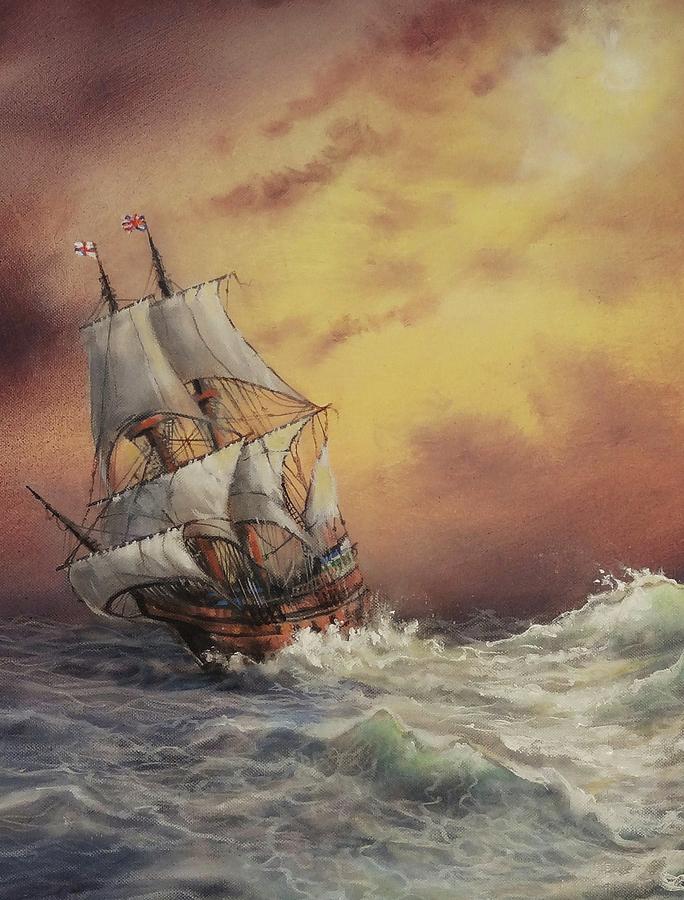The image, presented in a portrait orientation, appears to be a photograph of a painting depicting a tumultuous maritime scene. Dominating the foreground is a large wooden sailboat, reminiscent of a pirate ship, complete with two substantial masts adorned with a total of six white sails. The vessel, which bears a tiny British flag atop one of the masts and another flag on the other, is dramatically leaning to the left, as if on the verge of capsizing. It's being relentlessly tossed by the extremely rough, stormy seawater, with formidable waves crashing against its starboard side. The background is dominated by an ominous, dark, and very cloudy sky, casting a foreboding atmosphere over the scene, though a small burst of sunlight breaks through in the top right corner, adding a touch of contrast to the otherwise bleak setting.